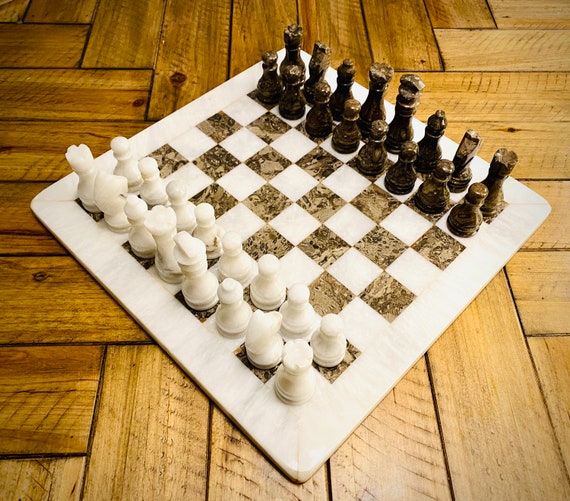The image depicts a luxurious chess set laid out on a wooden floor. The chessboard itself is crafted from an elegant, granite or marble material, with alternating white and dark brown squares, the latter featuring a slight marbled pattern. The board is tilted such that one corner points towards the bottom of the image, with the opposite corner pointing towards the top, and the remaining two corners directed to the left and right sides of the frame. The chess pieces, made from the same luxurious material as the board, are meticulously arranged with the white pieces in the foreground (left side) and the black pieces towards the background (upper left side). The wooden floor beneath the board consists of asymmetrical, interlocking panels that vary in tone, displaying a two-tone design that transitions from darker on the left to lighter on the right. The artificial lighting in the room casts subtle reflections off the glossy surface of the chessboard, enhancing the overall sophistication of the setup.